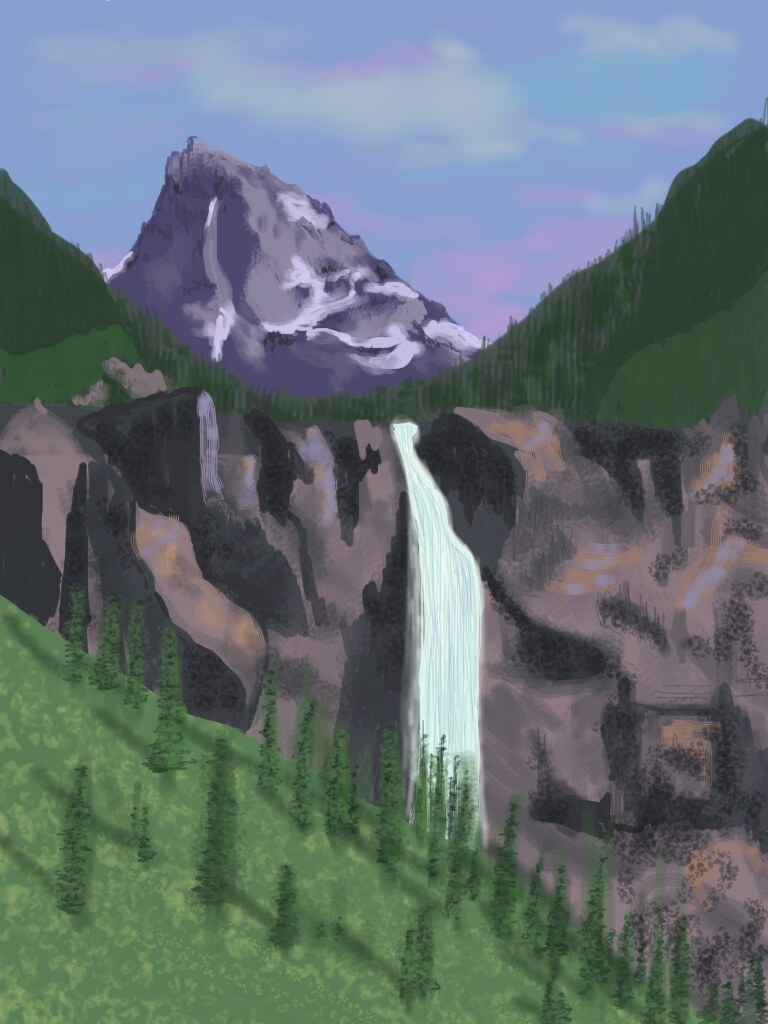This image depicts a vibrant and detailed landscape painting, likely created using digital or acrylic mediums. The top half of the composition features a sky painted in a periwinkle bluish-purple with splashes of pink and light blue. Subtle, fluffy white clouds add texture to the upper expanse. Below the sky, a stark, snow-dusted mountain peak rises prominently, composed solely of stone and rock with no vegetation. Surrounding this peak are verdant hills and cliffs, the latter appearing more brown in tone and featuring a mesmerizing waterfall cascading down their center. The grassy hills are accentuated by lighter strokes suggesting dense clusters of trees. In the bottom left corner, a green hill flourishes with visibly distinct pine trees, creating a rich, natural tapestry within the landscape.